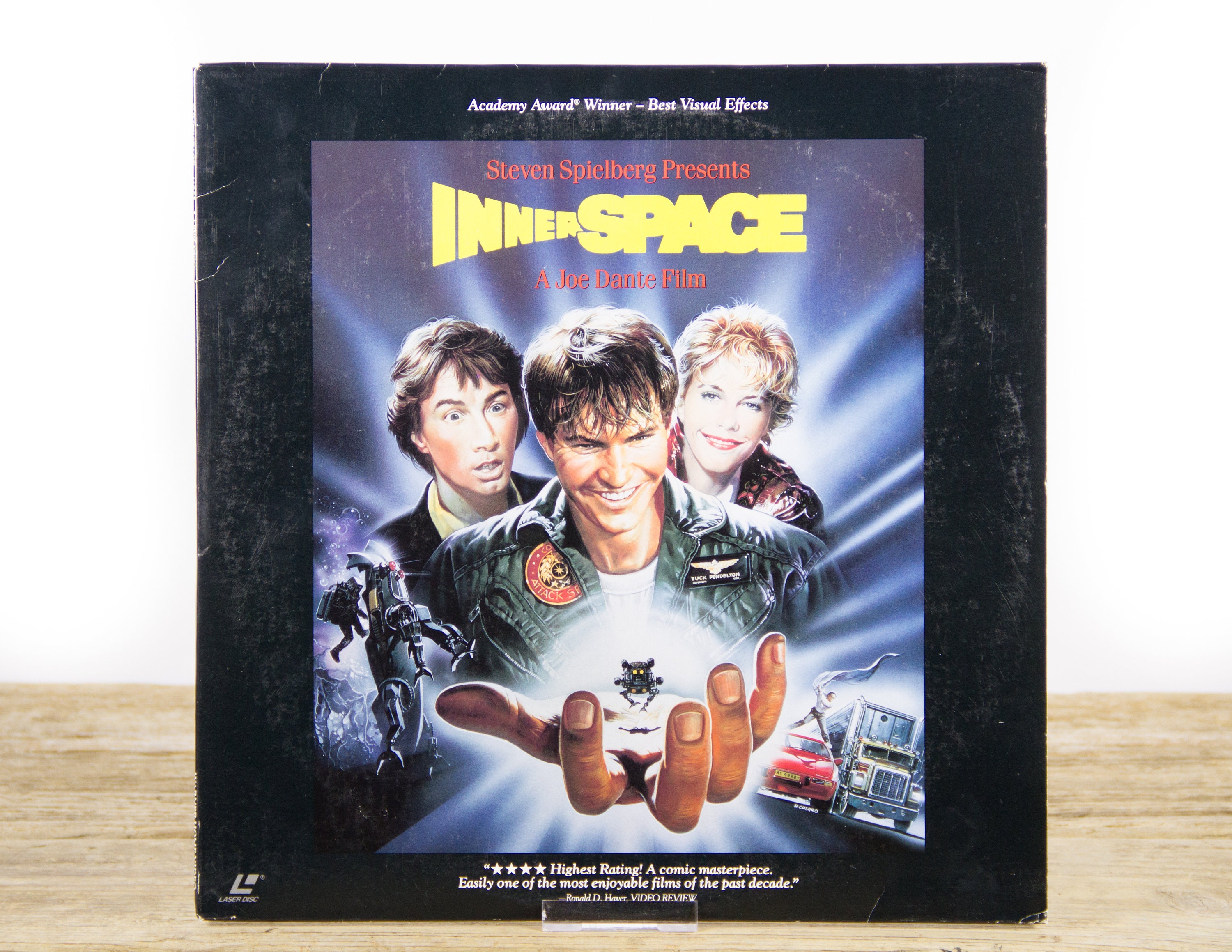This image is a detailed cover for the movie "Innerspace," presented by Steven Spielberg and directed by Joe Dante. Prominently displayed at the top is an accolade, "Academy Award winner for Best Visual Effects." The central photo on the cover features three actors, likely Martin Short, Meg Ryan, and another character in the middle who is possibly dressed in a space aviator type jacket with visible wings clipped on. All three are gazing in excitement at a crystal-clear bubble held by an invisible hand, inside which resides a peculiar robot-like creature, illuminated by a light. The background is a collage of vibrant scenes, including a partial view of the Earth, a figure floating in space, and another robot-like entity. Additionally, part of the background features a strip of light wood, a semi-truck, and a red sports car with someone standing on it. At the bottom, it highlights critical acclaim: "Four stars, highest rating, a comic masterpiece, easily one of the most enjoyable films of the past decade." The Laserdisc logo appears in the bottom left corner, confirming that this is a Laserdisc cover, a vintage form of media.